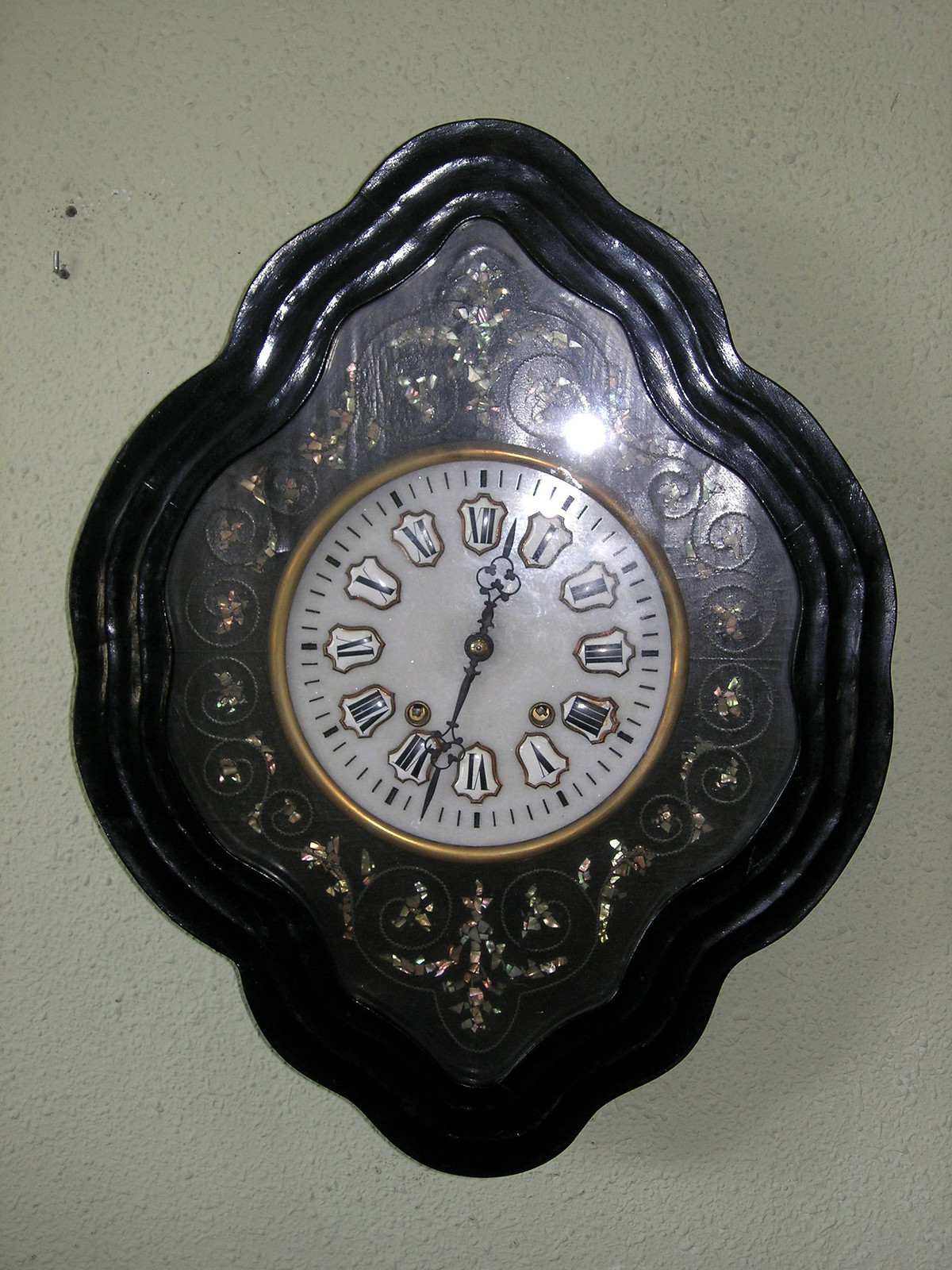On a textured white background, a clock face is centrally positioned. The clock features the traditional numbering with 12 at the top and 6 at the bottom, but interestingly, each number is set within a room-like section. Encircling the clock face are numerous dark dashes, prominently marked at each numeral. Reflections emanate from the clock, forming lines reminiscent of plant stems. These reflections create a striking black wave that extends towards the left and right sides of the clock. Additionally, the clock is adorned with intricate silver patterns, adding an elegant touch to its overall design.